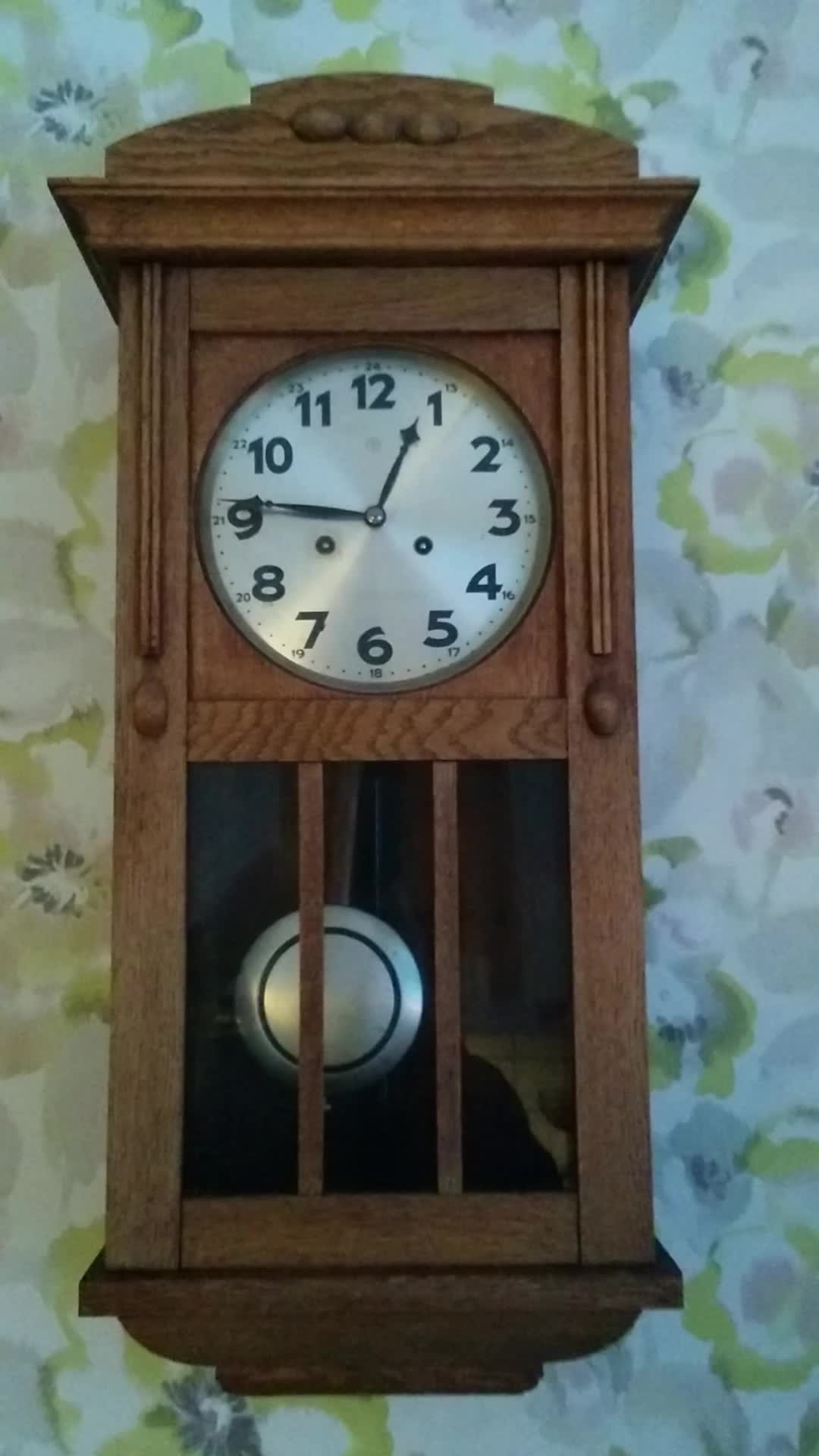The image depicts a detailed and elegantly crafted wall-mounted grandfather clock encased in a dark brown wooden cabinet. The clock's face is a silverish-gray color adorned with bold black numerals and black clock hands, indicating the time as 12:46, with the long hand on the 9 and the short hand near the 1. Below the clock face, there is an open section with a glass cover, featuring two vertical brown wooden strips that frame a visible silver pendulum. The background showcases a beautifully patterned wall, featuring light gray and greenish hues with delicate, watercolor-like floral designs that add an artistic touch to the serene white backdrop. At the top, the clock features a layered design that rises to a smaller point, adding a classic touch to its sophisticated appearance.